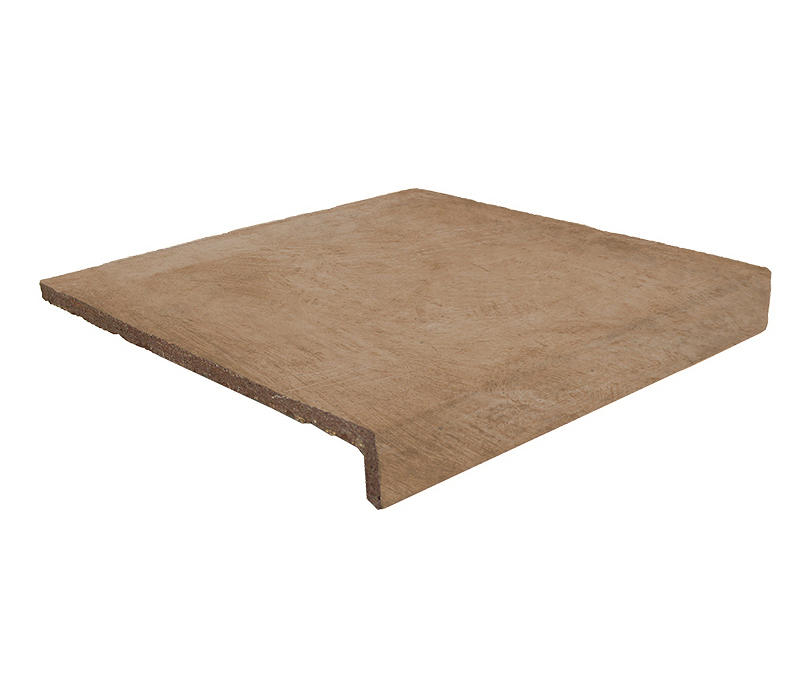The image depicts a plain, undecorated wooden panel seemingly made from cheap, recycled plywood, characterized by its brown hue and rough, uneven edge. This panel is viewed from a 45-degree angle, making it appear diamond-shaped. The panel features a downward-facing lip along its rightmost edge, resembling an inverted L shape. Notably, the wood shows scratch lines that do not shift directions to follow the lip, raising questions about potential image editing or the material's inherent texture. Set against an empty white background, the panel floats without any discernible support, giving it an isolated, product-photo appearance typical of online listings for construction materials, like flooring or cabinet panels.